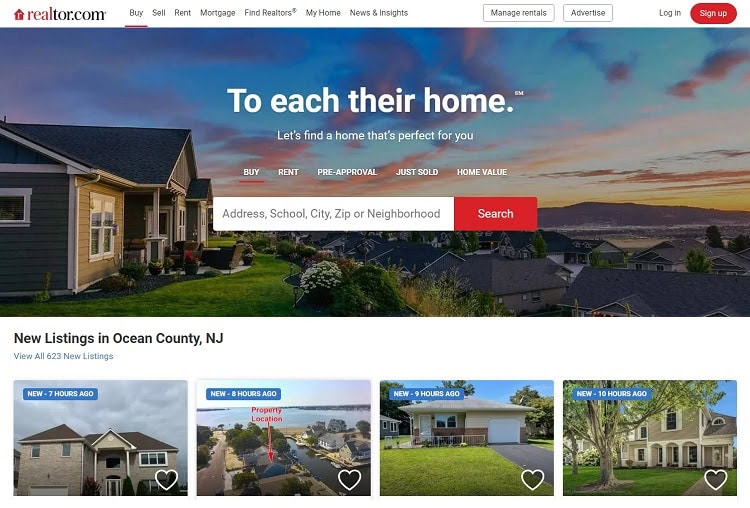This image is a screenshot from the website Realtor.com. At the top of the page, the logo features "realtor" in red and ".com" in black with a white background. Below the logo, there is a navigation bar with the following headings: "Buy," "Sell," "Rent," "Mortgage," "Find Realtors," "My Home," "News & Insights." Additionally, there are bordered areas labeled "Manage Rentals" and "Advertise." To the far right, "Log In" and "Sign Up" options are available, with the "Sign Up" button prominently highlighted in a red circle with white text.

The main banner, set outdoors, depicts a house to the left under a blue sky scattered with pink and white clouds. Below this, a mountain range forms the backdrop of a picturesque neighborhood. Bold text reads, "To reach their home," accompanied by finer print stating, "Let's find a home that's perfect for you."

Further down, options labeled "Buy," "Rent," "Pre-Approval," "Just Sold," and "Home Value" are displayed alongside a search bar prompting users to enter an "Address, School, City, Zip, or Neighborhood." A red search button with white text is adjacent to this input field. Underneath, the site highlights "New Listings in Ocean City or Ocean County, New Jersey" in black text, with a clickable option to "View all 623 listings." Below this, there are thumbnail images of four different homes available for sale.